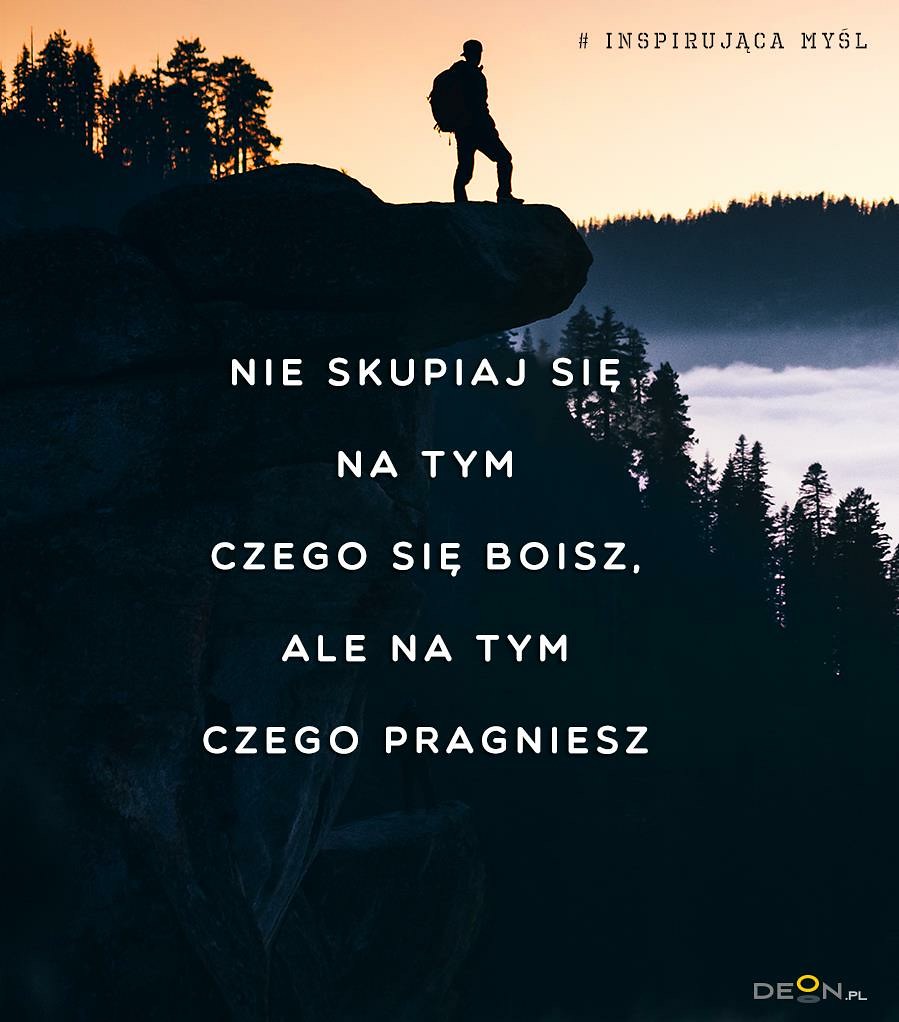The image depicts a solitary hiker, a man dressed in typical hiking attire — a backpack, a backwards cap, cargo shorts, and hiking boots — standing on the edge of a cliff. His silhouette, dark and defined, contrasts sharply against the serene, peach-colored sky, suggesting either a sunrise or sunset. He gazes out over a sweeping, expansive view that includes densely forested areas both at the bottom of the cliff and in the distant background. The sky is bathed in soft, warm hues of orange, with a white glow illuminating the tops of distant trees, possibly pine trees. The scene is imbued with a tranquil atmosphere. An inscription in a foreign language runs across the middle of the image, adding an element of intrigue, while the bottom right corner features a logo that reads "DEON.PL." This striking image may serve as a poster promoting outdoor adventure and the beauty of nature.